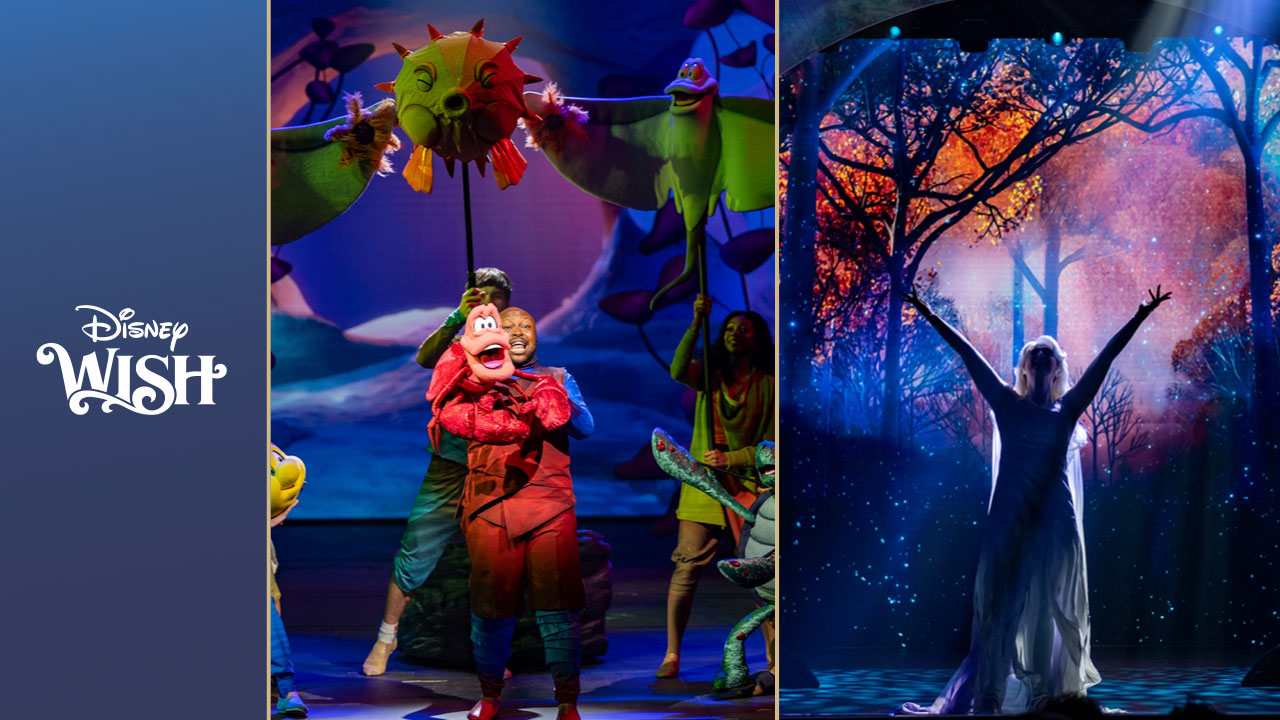The image consists of two photographs from a Disney Wish cruise brochure showcasing live stage performances. On the right, a woman in a white dress stands on a dimly lit stage, her arms raised towards the sky. The backdrop features trees and speckles of light, reminiscent of snow, creating an enchanting, somewhat ethereal ambiance. This scene likely represents an Elsa performance from the Frozen series, characterized by its forest scenery and sparkling lights. On the left, the stage is animated with characters holding various puppets and images of fish, and a singer dressed as a crab. This lively depiction, filled with oceanic elements, suggests a scene from The Little Mermaid, possibly featuring puppetry. The left side of the image prominently displays the Disney Wish branding, underscoring the cruise's theme of immersive Disney theatrical experiences.